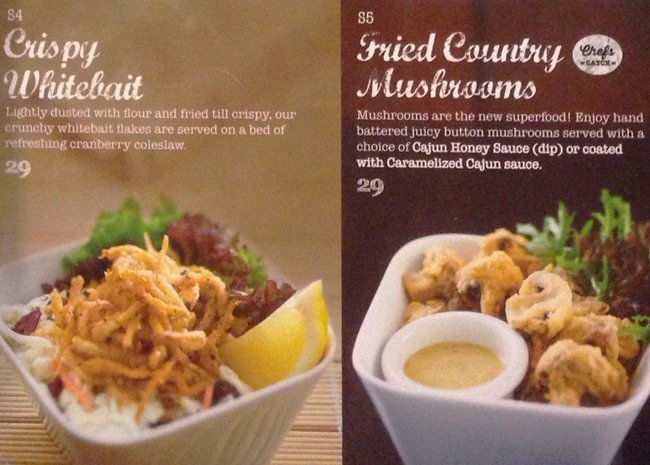The image appears to be from a recipe book or a food magazine, displaying two enticing dishes, each in its own white rectangular boat against a visually appealing background. The left side titled "S4 - Crispy White Bait" features flaky, lightly dusted, and crisply fried white bait served on a refreshing bed of cranberry coleslaw, accompanied by a lemon wedge and brown and green vegetable garnishes. The right side titled "S5 - Fried Country Mushrooms" showcases hand-battered juicy button mushrooms, hailed as the new superfood, with an option of Cajun honey sauce dip or a coating of caramelized Cajun sauce. Both sides contain detailed images of the respective dishes, highlighting their texture and presentation, with the left side presented on a darker, earthy-toned surface and the right side emphasizing vibrant, contrasting tones.